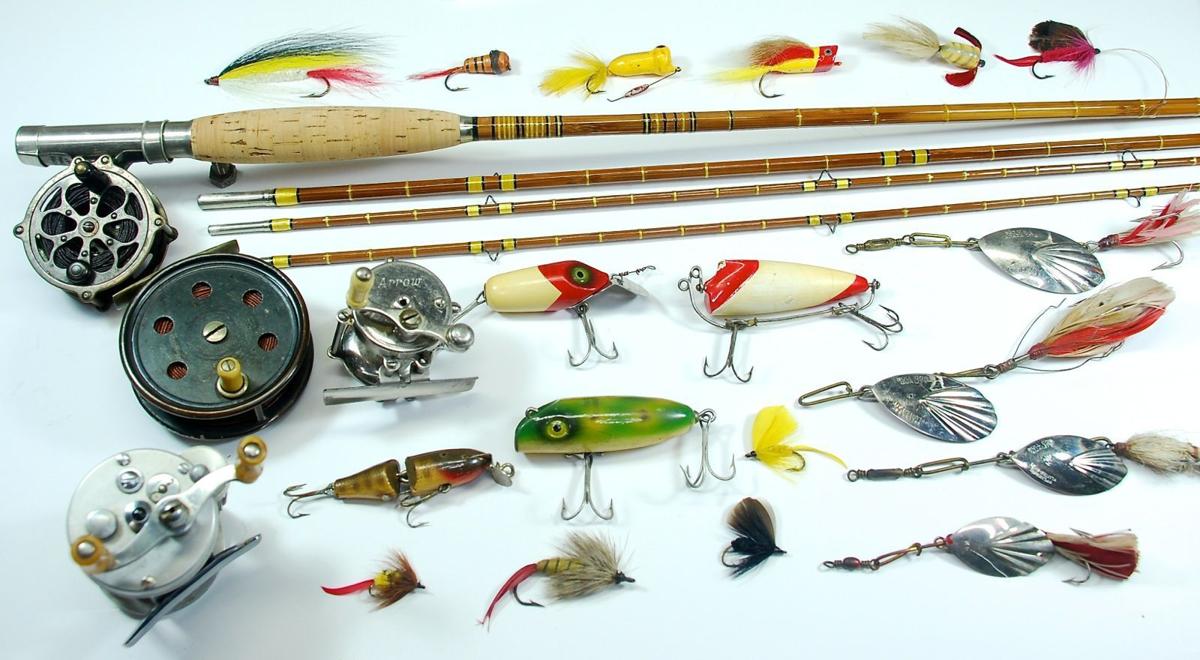This image showcases a meticulously arranged collection of vintage fishing equipment against a white background. Centrally featured is a broken-down fishing rod in four sections, likely bamboo or a dark oak color, with a handle made of cork displaying brown with yellow stripes. To the left of the rod is a deconstructed reel in silver, black, and white, that appears to be in excellent, possibly restored, condition. Six intricately detailed fly-fishing lures with feathery tails are aligned at the top, while various other lures and bobbers – including fish-like, feathered, and metallic ones – are spread across the bottom of the display. The strategic layout of these items, which also includes spinning spindles and additional reels in similar silver hues, suggests this may be a presentation for a fishing site or a museum exhibit, rather than a sales platform.